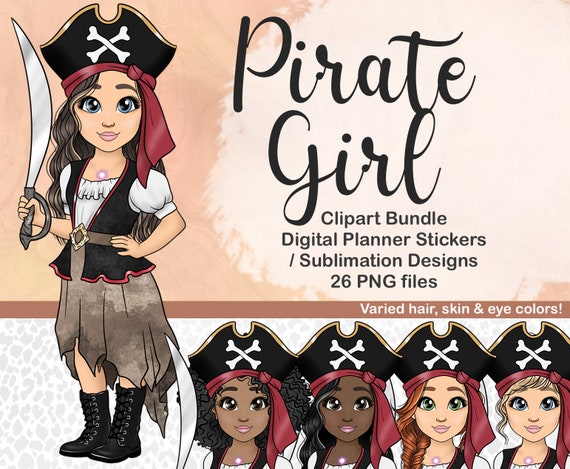This detailed infographic, designed as a digital advertisement, showcases a collection of vibrant clip art of pirate girls. The page is divided with a background that transitions from tan on top to light gray and white below. Centrally, the title "Pirate Girl" appears in cursive against a light tan backdrop, followed by the description: "Clip Art Bundle, Digital Planner Stickers, Sublimation Designs, 26 PNG Files." A brown bar stretches across the graphic, declaring in white text, "Varied Hair, Skin, and Eye Colors."

Prominently featured on the right is a full-body illustration of a pirate girl with pale skin and expressive blue eyes. She dons a black pirate hat adorned with crossbones and a red bandana beneath it. Her brown hair cascades down, and she wields a sword in her right hand, which is bent at the elbow. She wears a pink necklace, a ruffled short-sleeve pirate shirt, a black vest, a belt, and a tattered brown skirt. Her ensemble is completed with mid-calf black tie-up boots.

At the bottom left, four additional pirate girls display the advertised variations in appearance. The first girl has caramel skin and dark curly hair. Next is a darker-skinned girl with wavy black hair. The third has pale skin and red hair with greenish eyes, and the fourth is even paler with blonde hair and blue eyes. Each character is depicted from the shoulders up, emphasizing the diverse range of hair, skin, and eye colors available in this clip art bundle.